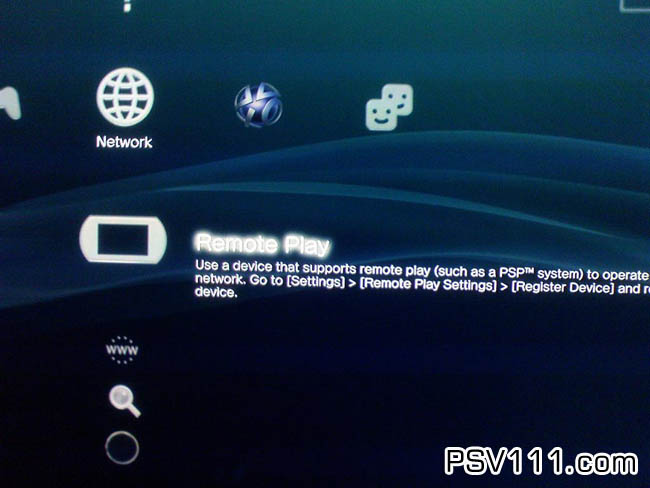The image appears to be a screenshot capturing the infotainment center of a vehicle's screen, or potentially a smart TV or computer display. The dominant colors are various shades of blue, accented with white highlights. The background features a dark blue and black wave pattern, with turquoise highlights that create a serene, fluid aesthetic. A central image showcases a globe icon labeled "network," indicating internet connectivity options. Next to this icon are another symbol and two overlapping squares with smiley faces.

Prominently displayed in the center is a text block that reads "Remote Play," with instructions below that advise, "Use a device that supports remote play, such as a PSP system. PSP is a trademark symbol." The detailed steps provided include navigating to "Settings," selecting "Remote Play Settings," and choosing "Register Device." The word "and" is followed by a partially obscured word starting with "R," likely cut off in the image, and then the word "device" again appears.

Additional icons below these instructions include a "www" within a circular icon, suggesting a web link, and a magnifying glass symbol indicating a search function. In the lower right corner, the text "psv111.com" is visible, hinting at a web address or specific connectivity interface related to the image's content. There are no people in the picture, and all visual elements contribute to a cohesive and technology-focused theme.